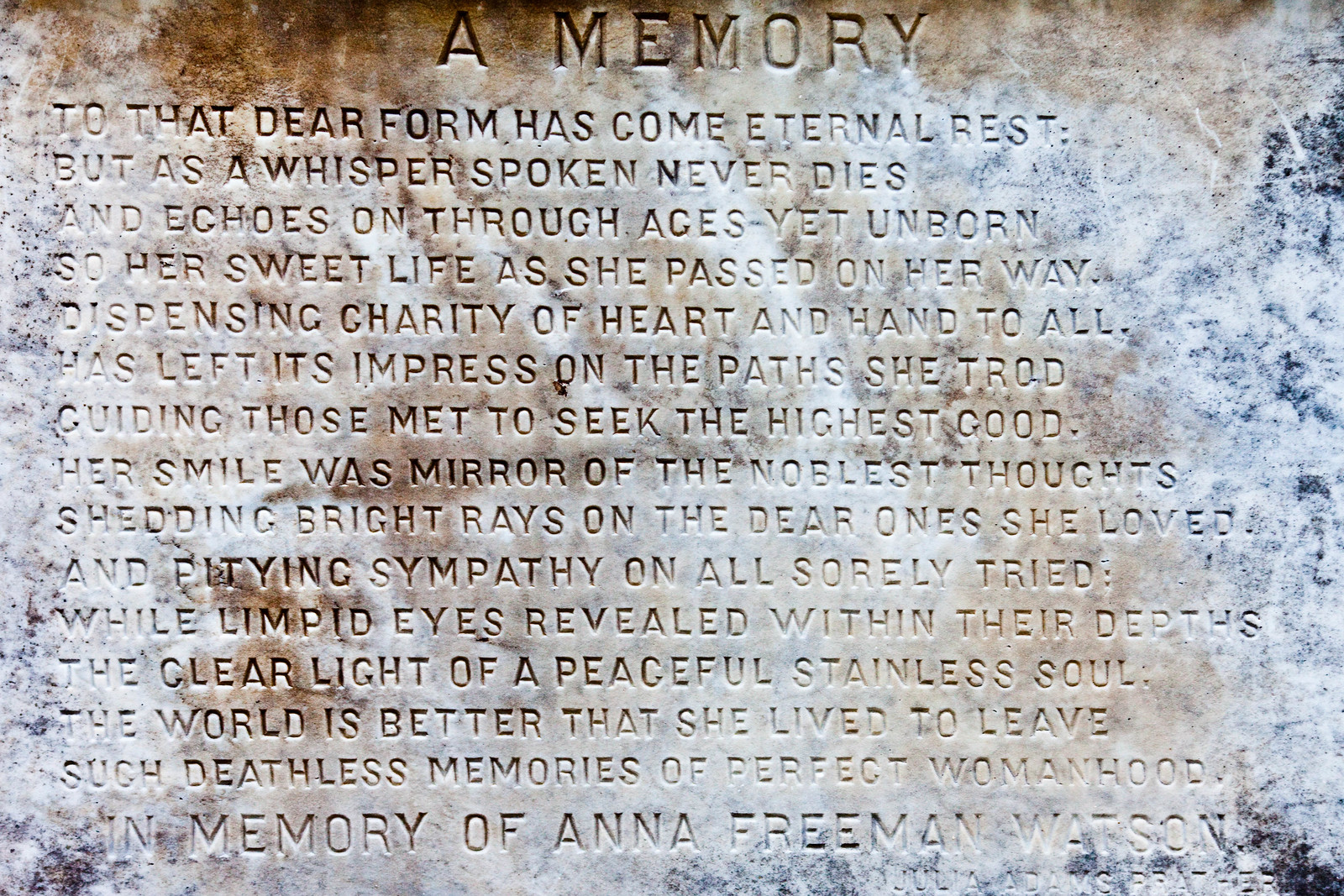The image depicts an old, weathered gravestone of brownish-stained marble, featuring an elaborate inscription dedicated to Anna Freeman Watson. At the top of the gravestone, in a formal font, are the words "A Memory." Below this heading is an intricately etched poem that pays tribute to Anna, reflecting on her eternal rest and her life that had a lasting impact on others. The poem honors Anna’s virtues, such as her charity, noble thoughts, and serene soul, suggesting she dispensed kindness and left a significant impression on those around her. The gravestone likely has a large base, suggesting its significance and the care taken to commemorate Anna. The text highlights that her legacy of perfect womanhood and eternal memories continues to inspire.